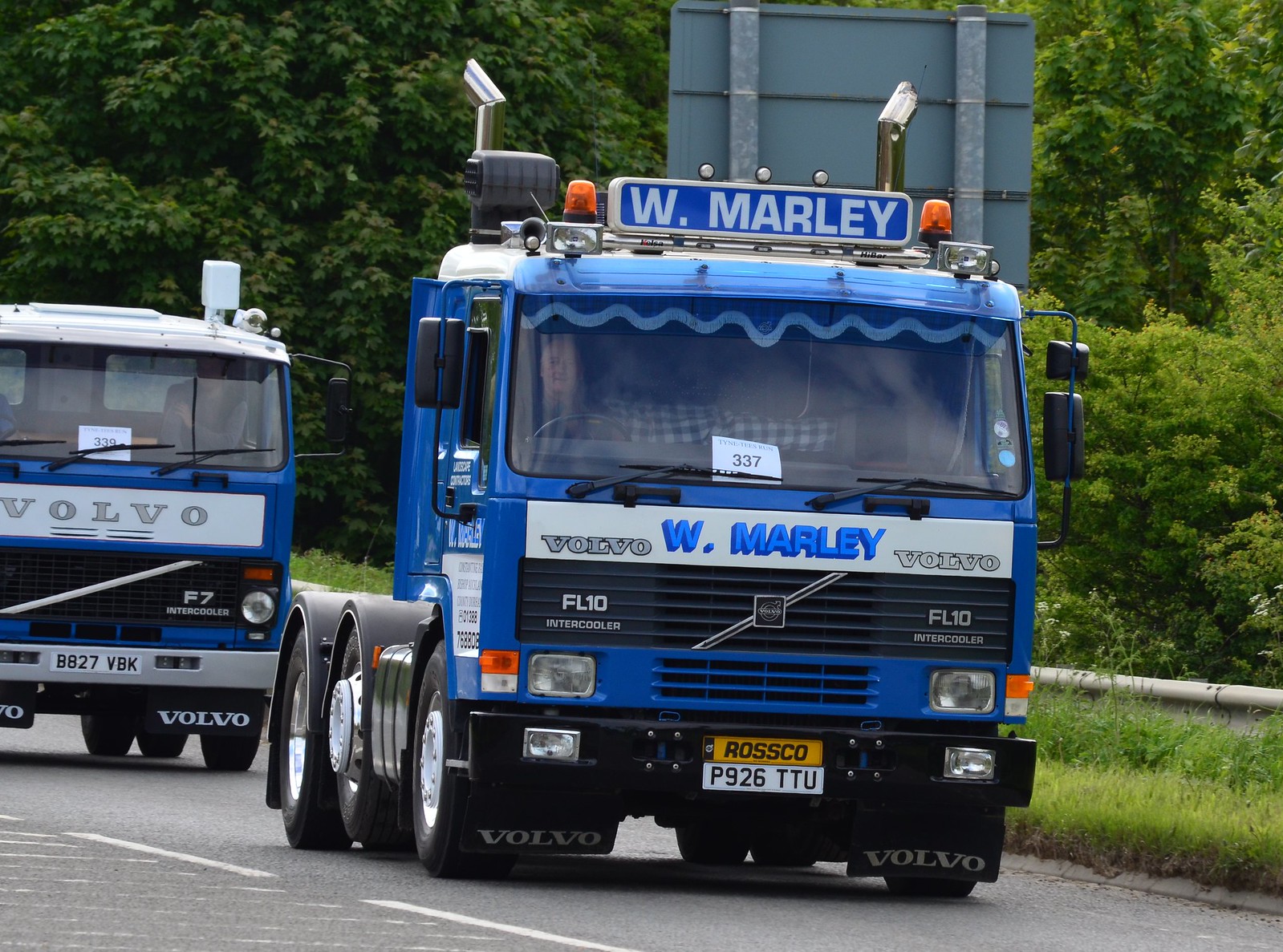The image depicts two semi-tractor trailer trucks, both without trailers, situated on a road bordered by green grass and tall, leafy trees in the background. The trucks appear to be parked or driving on what seems to be a highway, marked by a grey brick edging separating the road from the grassy areas.

The truck in the front is primarily blue with a white front section that features intricate detailing. On the white portion, "Volvo" is prominently displayed in silver on both the right and left sides. In the center of this section, "W. Marley" is written in blue, and beneath that, it reads "FL 10 intercooler." The vehicle's license plate, displayed in white with black text, reads "P926TTU," and above it, there's a gold emblem with the name "Rosco." This truck also features large, robust tires, Volvo mudguards, and visible smokestacks.

Following closely behind is another truck, predominantly white with blue accents. This second vehicle also has "Volvo" emblazoned on its front, above the designation "F7 intercooler." Through the windshields, one can discern some dashboard details and possibly paperwork with numbers. The two trucks share a similar make and color scheme, suggesting they may belong to the same fleet or company. The backdrop is filled with verdant trees, and a clear road occupies the lower portion of the image.